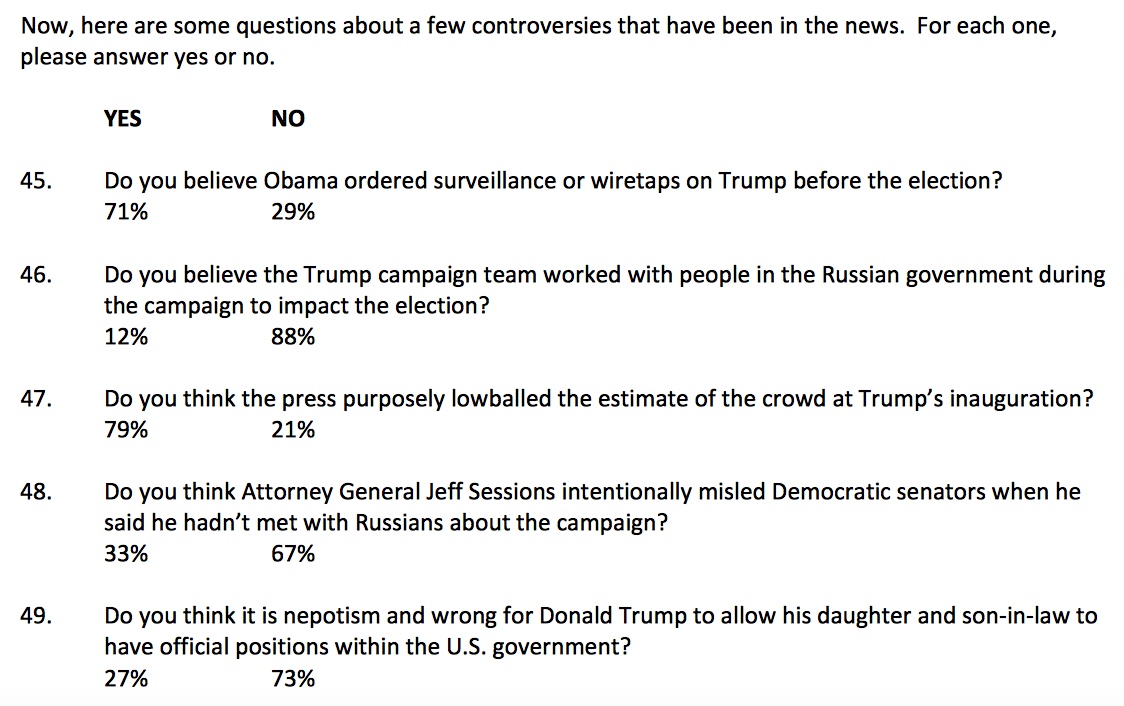This image is a cropped screenshot of a quiz addressing current controversies, instructing participants to answer each question with either "yes" or "no." At the top, it states, "Now here are some questions about a few controversies that have been in the news. For each one answer yes or no." 

The left side shows the percentage of "yes" responses, while the right side shows the percentage of "no" responses. The screenshot captures questions numbered 45 to 49. 

1. **Question 45:** "Do you believe Obama ordered surveillance or wiretaps on Trump before the election?" — 71% responded "yes," and 29% responded "no."
2. **Question 46:** "Do you believe the Trump campaign team worked with people in the Russian government during the campaign to impact the election?" — 12% responded "yes," and 88% responded "no."
3. **Question 47:** "Do you think the press purposely lowballed the estimate of the crowd at Trump's inauguration?" — 79% responded "yes," and 21% responded "no."
4. **Question 48:** "Do you think Attorney General Jeff Sessions intentionally misled Democratic senators when he said he hadn't met with the Russians about the campaign?" — 33% responded "yes," and 67% responded "no."
5. **Question 49:** "Do you think that it is nepotism and wrong for Donald Trump to allow his daughter and son-in-law to have official positions within the US government?" — 27% responded "yes," and 73% responded "no."

Each percentage closely reflects the public's stance on these issues, offering a glimpse into the prevailing opinions during the time the quiz was taken.